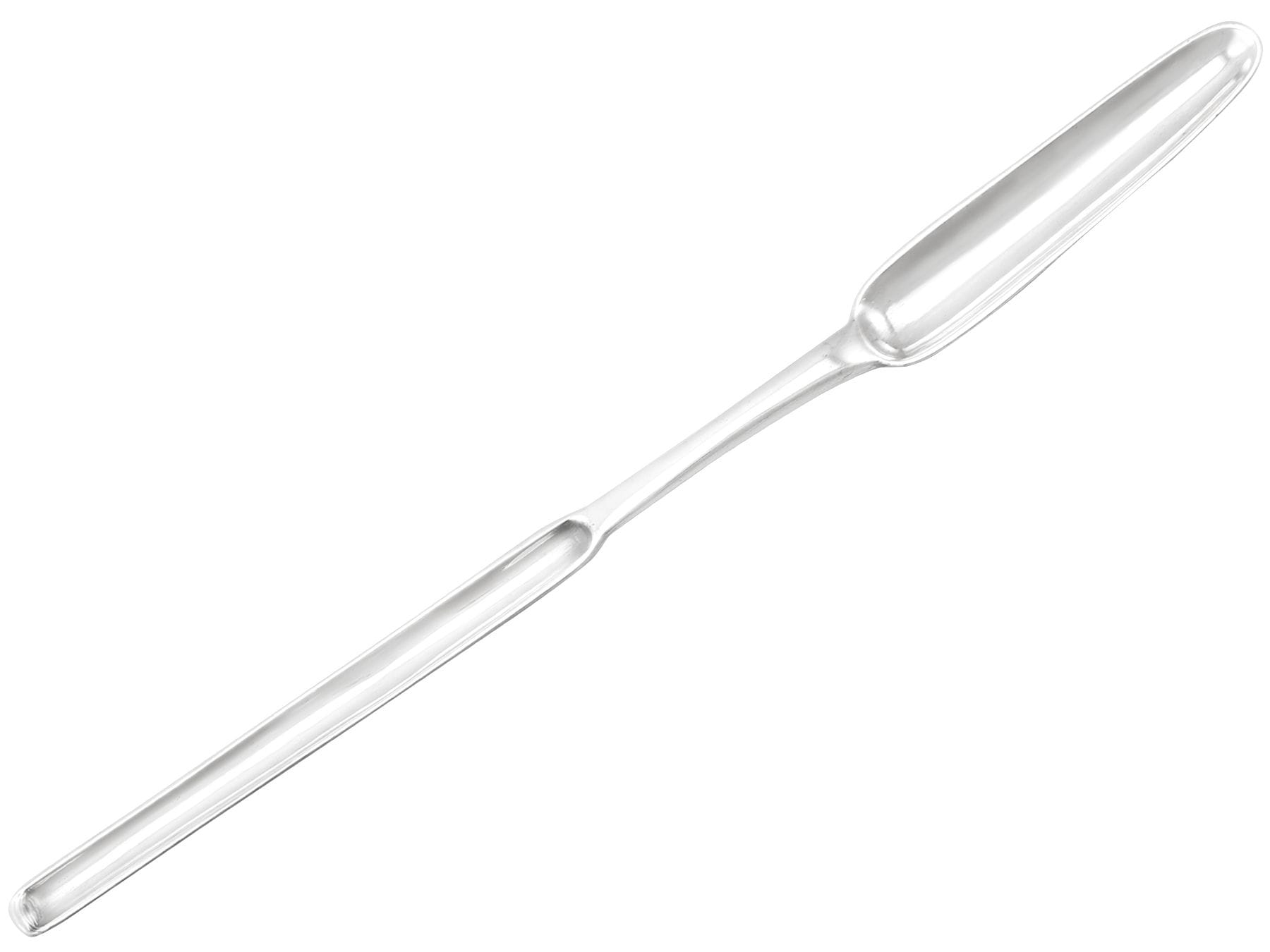The image depicts a highly polished, reflective silver utensil, resembling a slender, elongated spoon or possibly a medical device, set against a completely white background. The object is diagonally positioned with the narrow end pointing towards the upper right corner and the back end directed towards the bottom left. The utensil, which might be a marrow scoop or a tool for extracting meat from crabs, features a very shallow, long scoop at one end, a flat midsection, and a slightly broader, spoon-like portion at the other end. The minimalist setting enhances the professional presentation of the well-crafted, thin, and delicate-looking utensil.